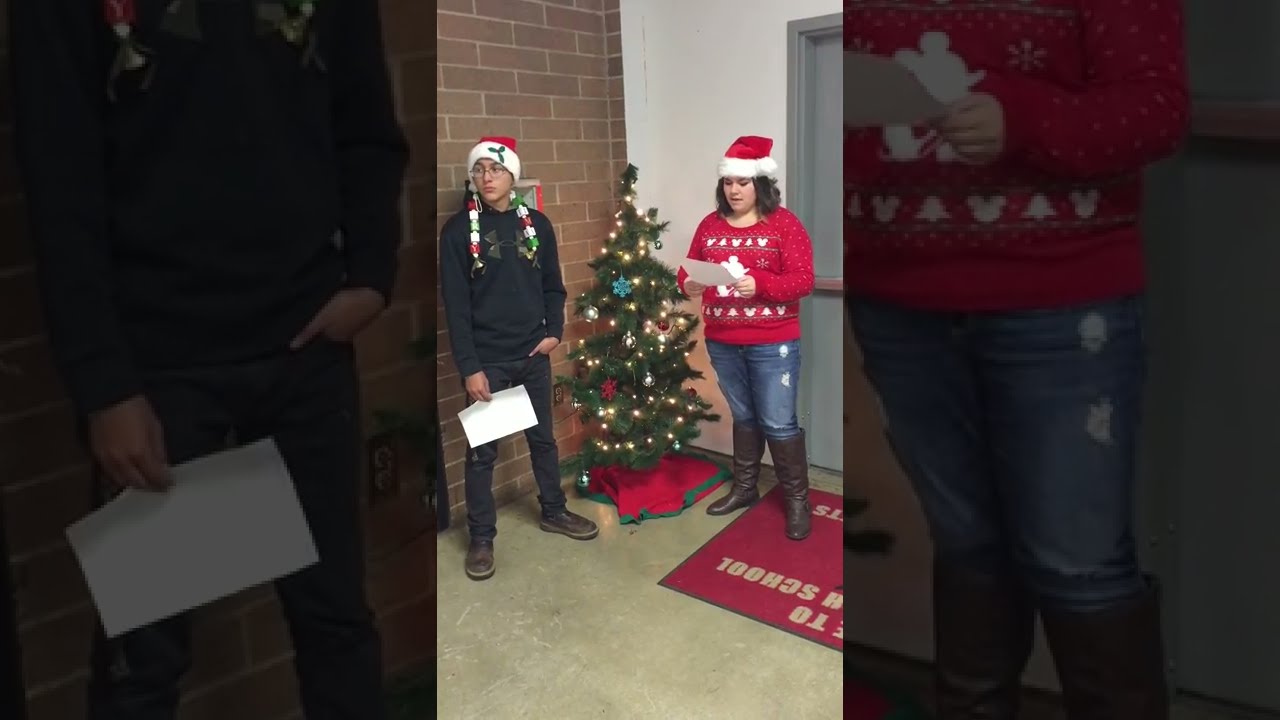In this indoor photograph taken in a school hall, likely a corner with a white wall on one side and brown-bricked wall on the other, two teenagers are the focal point, flanking a festively decorated Christmas tree. The tree, about four feet tall, stands adorned with blue and red snowflake ornaments, entwined with bright white lights and wrapped in a red tree skirt with green trim. To the left of the Christmas tree is a teenage boy with light brown skin. He wears a Santa hat adorned with a holly leaf and berries on the white brim, a long-sleeved black Under Armour hoodie, black jeans, and brown boots. Around his neck, a block-style Christmas decoration with bronze bells dangles, and he looks down at a piece of paper in his right hand while his left hand rests in his pocket. On the right side of the tree stands a Caucasian girl with shoulder-length brown hair, also in a Santa hat. She wears a red long-sleeved sweater featuring a Mickey Mouse Christmas design, blue distressed jeans, and knee-high brown boots. She too is engrossed in a piece of paper held with both hands. The floor beneath them is shiny linoleum, leading to a red rug in the lower right-hand corner, which bears text referencing the school. The setting, festive attire, and decorations suggest a Christmas celebration event at the school.